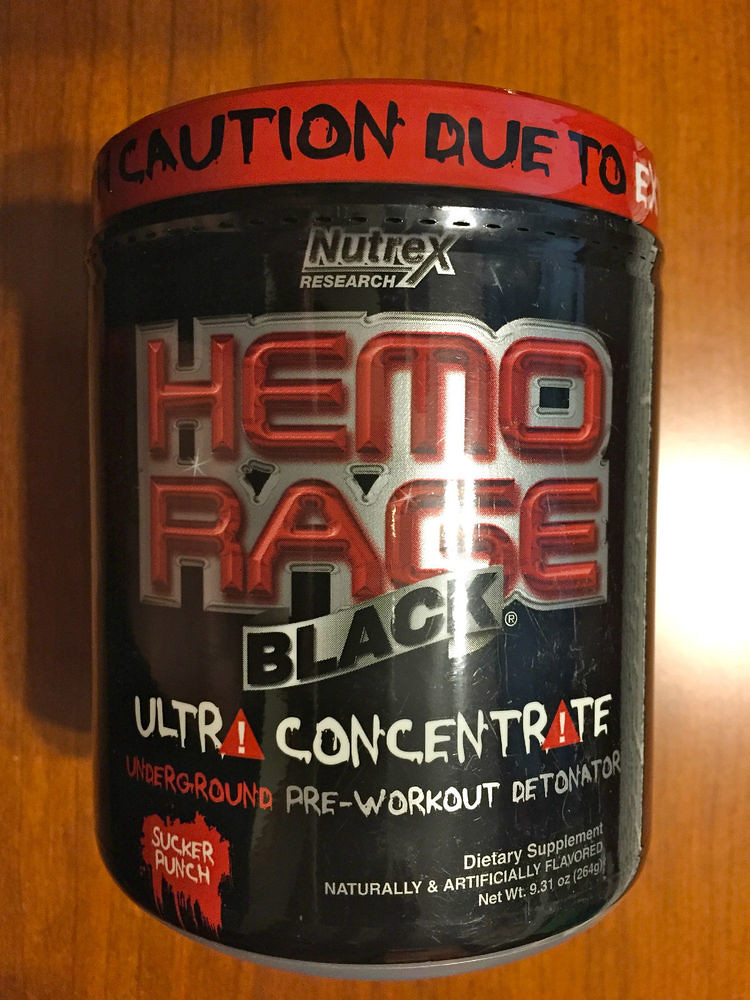This is an artist's rendition featuring a hyper-realistic mixed-media artwork on a brown laminate wood table. The artwork appears to intricately blend painting with digital elements, creating a visually striking composition. The centerpiece of the image is a highly detailed depiction of a black container with a red lid, prominently marked with the word "Caution" followed by the partially obscured text "due to EX". 

The container displays the brand name "Nutrex" in capital letters, followed by "Research". Below that, in large block letters, is the product name "Hemo Rage" with another line underneath stating "Black" in matching black letters. Further down, the label reads "Ultra Concentrate" accompanied by two red triangular warning symbols with white exclamation points inside them. The text below identifies the product as an "Underground Pre-Workout Detonator".

In the bottom left corner of the container's label, the words "Sucker Punch" are written in white, accented with red paint-like splotches. Adjacent to this, additional text describes the product as a "Dietary Supplement, Naturally and Artificially Flavored", with a net weight of 9.31 ounces.